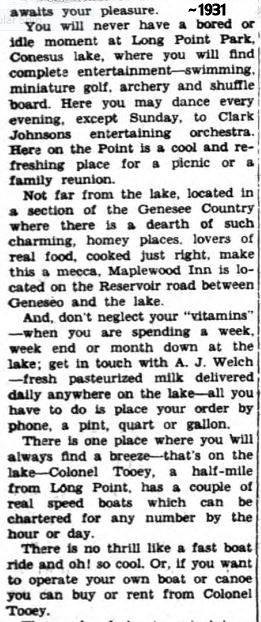This black-and-white image features an old newspaper clipping from 1931. The clipping, densely packed with fine print, describes various recreational opportunities at Long Point Park on Conesus Lake, promising "complete entertainment" including swimming, miniature golf, archery, and shuffleboard. The article emphasizes evening dances, held every night except Sunday, to the music of Clark Johnson's entertaining orchestra. Known for its refreshing and picturesque ambiance, the spot is ideal for family picnics and reunions. Nearby is the Maplewood Inn on Reservoir Road, between Geneseo and the lake, highlighted as a culinary haven amidst an area scarce in charming homing places. The article also mentions fresh pasteurized milk, delivered daily by A.J. Welch, available by phone order in various quantities. Additionally, Colonel Tuohy offers the excitement of speedboat rides a half-mile from Long Point, with options to charter or rent boats and canoes. The composition of the image focuses solely on the printed words, capturing the essence of an era teeming with vibrant community activities and wholesome fun.